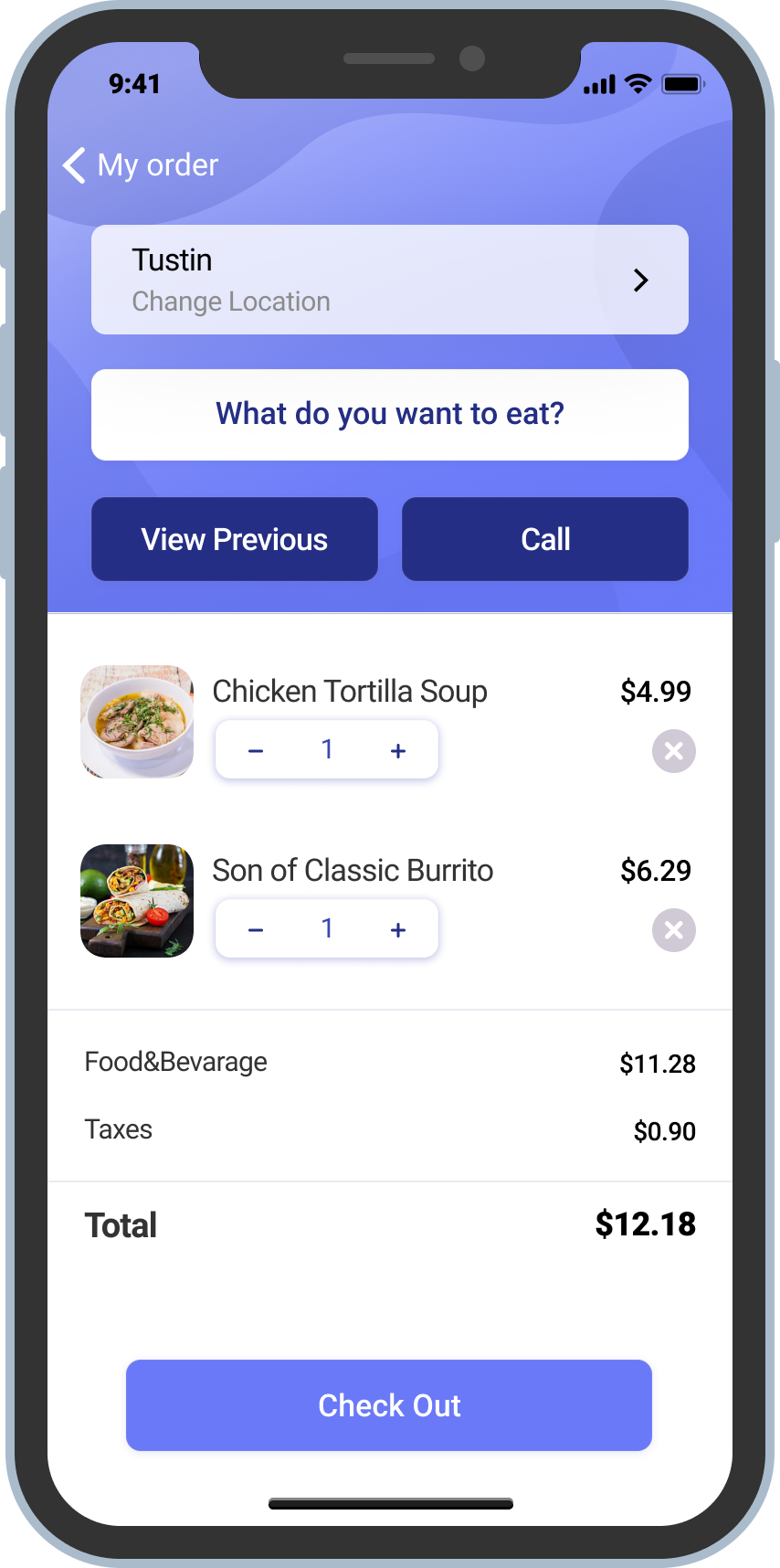The image is a screenshot taken on a mobile phone, depicting an online food ordering interface. The top section of the screen features a purple background with several elements: a title "My Order" indicating the location as "Tustin" with an option to change it. Below this, prominent navy-blue buttons labeled "View Previous" and "Call" are visible.

Underneath, the screen lists menu items: "Chicken Tortilla Soup" priced at $4.99, and "Son of Classic Burrito" priced at $6.29. The subtotal for food and beverages is noted as $11.28, with taxes amounting to $0.90, bringing the total to $12.18.

At the very bottom, there's a large, periwinkle-colored checkout button with the word "Checkout" written in white. 

The top status bar shows the time as 9:41 on the left side, and on the right side, it displays connectivity icons: black signal bars, the Wi-Fi symbol, and a fully charged battery icon also in black.